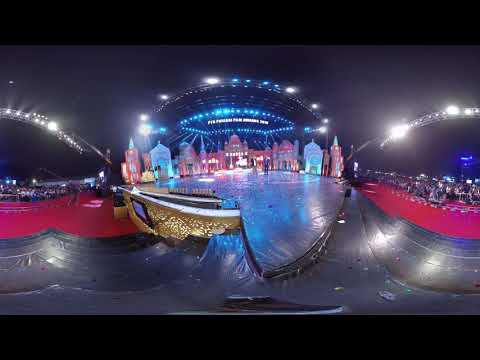This horizontally-aligned rectangular image, framed by thick black borders at the top and bottom, depicts a panoramic and somewhat distorted view of a vibrant event stage, likely a performance or concert. The center of the image features a colorful and elaborate set resembling a blue and red castle, possibly serving as an entrance to a theme park. Circular patterns of bright lights, predominantly blue, illuminate the scene from above, creating a festive atmosphere. The foreground showcases a wavy, gray-ground pattern, flanked by red carpeting on both the left and right sides. This red carpet extends beneath what appears to be audience seating, with crowds gathered behind railings, although their details are difficult to discern. The stage itself is empty, but its backdrop includes intricate, colorful set pieces that evoke miniature buildings or statues. Despite the slight blur and fisheye effect, the image captures the grandeur and excitement of the venue, highlighting the colorful lighting and detailed set design.